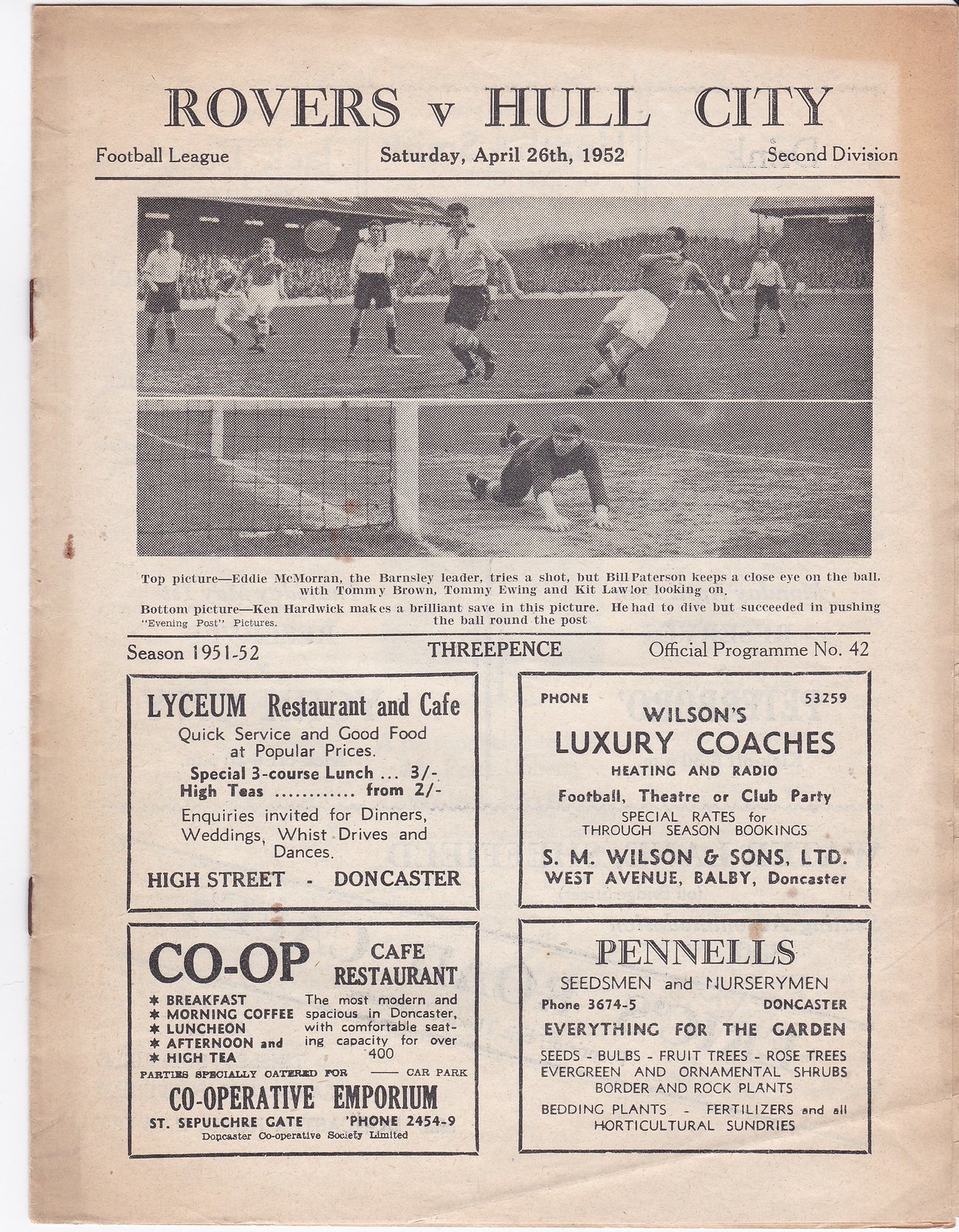The image depicts the cover page of a vintage soccer program from a match between Rovers and Hull City in the Football League's Second Division, dated Saturday, April 26, 1952. The background of the page is a soft, muted pink, reflecting its age as the paper has yellowed over time. The title at the top reads "Rovers vs. Hull City, Football League, Saturday April 26, 1952, Second Division," defining the event's historical context. 

The upper third of the page is occupied by black-and-white photographs capturing an intense football match, with notable action shots such as a goalie diving, albeit the ball is not visible. The program is identified as the official program number 42 for the season 1951-1952.

In the lower third, the page features two columns of advertisements. The left column includes an ad for the Lyceum Restaurant and Café, located on High Street in Doncaster, followed by an ad for the Co-op Café Restaurant at Sepulchre Gate. The right column contains an advertisement for Wilson's Luxury Coaches, offering services for football, theater, and club parties with special rates for groups. Below it is an ad for Penhalls, Seedsmen, and Nurserymen, also located in Doncaster, promoting gardening supplies. The program was priced at three pence, symbolized as 3p. 

This soccer program is a charming artifact from the mid-20th century, giving a glimpse into the sports culture and local businesses of the era.